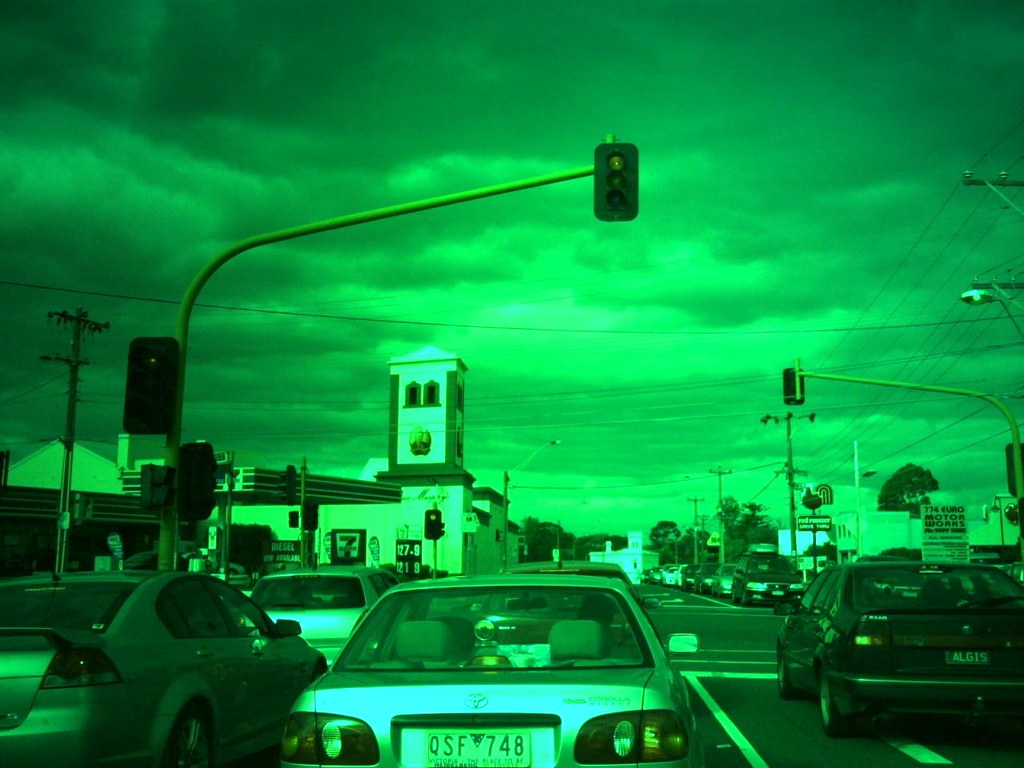The photograph features a vibrant dark green tint, likely the result of a filter, as seen in the tinted sky, clouds, vehicles, and surroundings. The image is taken from inside a moving vehicle, and in front of this vehicle is a silver car with the license plate QSF-748, bearing a silver Toyota symbol. The scene captures a busy street intersection with two traffic poles; each pole holds two traffic lights positioned overhead and at the edge, all showing red lights. While the cars and buildings on both sides of the street also bear the green tint, specific details like buildings on the left and right, a long line of cars, and a gas station are identifiable. The sky appears overcast, filled with dark green-tinted clouds and a centrally located sun.